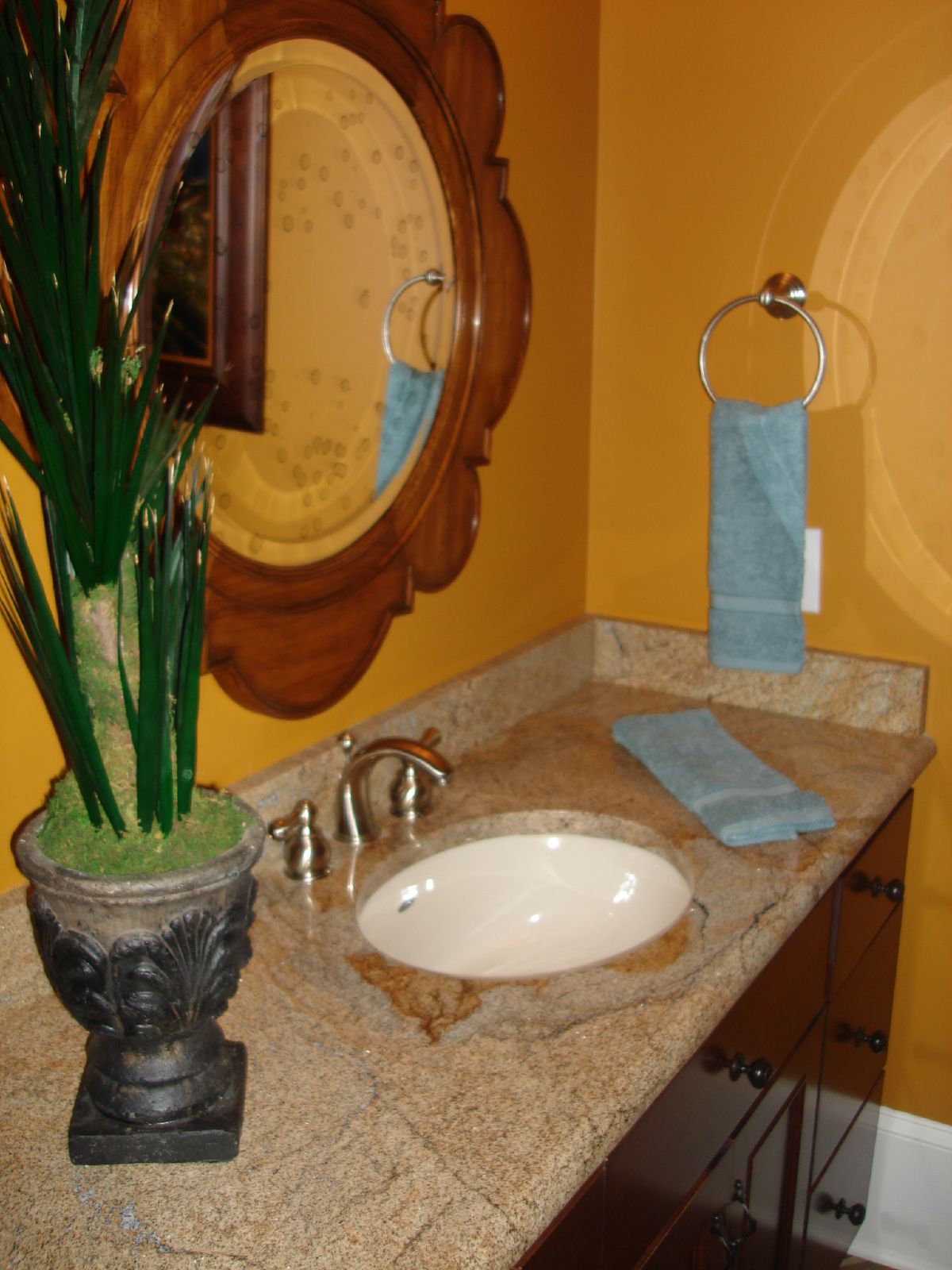This photograph features an elegantly designed bathroom sink counter. Dominating the space is a large, slightly oval-shaped mirror framed with dark wood, styled to resemble sun rays or flower petals. The rich, dark brown frame contrasts beautifully with the warm, orange-yellow wall behind it. The countertop is crafted from stone, showcasing a smooth blend of gray, orange, and white hues. Chrome fixtures adorn the sink, adding a touch of modern sophistication. A striking black planter sits on the counter, housing a vibrant cactus with sharp, sword-like green leaves. Completing the scene are two blue towels—one neatly hanging on a silver ring mounted to the wall, and the other laid out on the stone countertop.